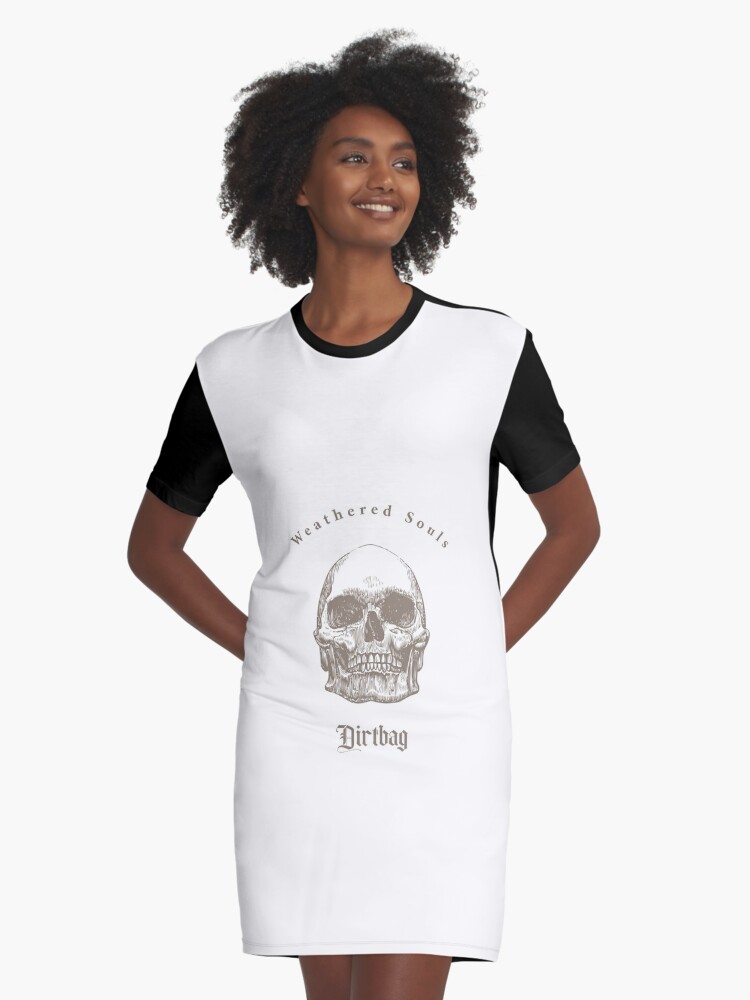The advertisement photograph features a tall African-descendant model, likely Ethiopian or Somalian, set against a completely white background. She stands in the foreground, centered, with her hands behind her back and her elbows pointing outward. Her tightly coiled, curly Afro hair frames her smiling face as she gazes off to her left. She is wearing a short-sleeved dress that reaches mid-thigh, detailed with black sleeves, a black neckline, and possibly a black back. The dress prominently displays the phrase "Weathered Souls" across the abdomen area, followed by a graphic of a skull and the word "Dirtbag" beneath it. The model's relaxed pose and vibrant smile add an air of carefree elegance to the image, making this an intriguing and visually compelling advertisement for the clothing retailer.